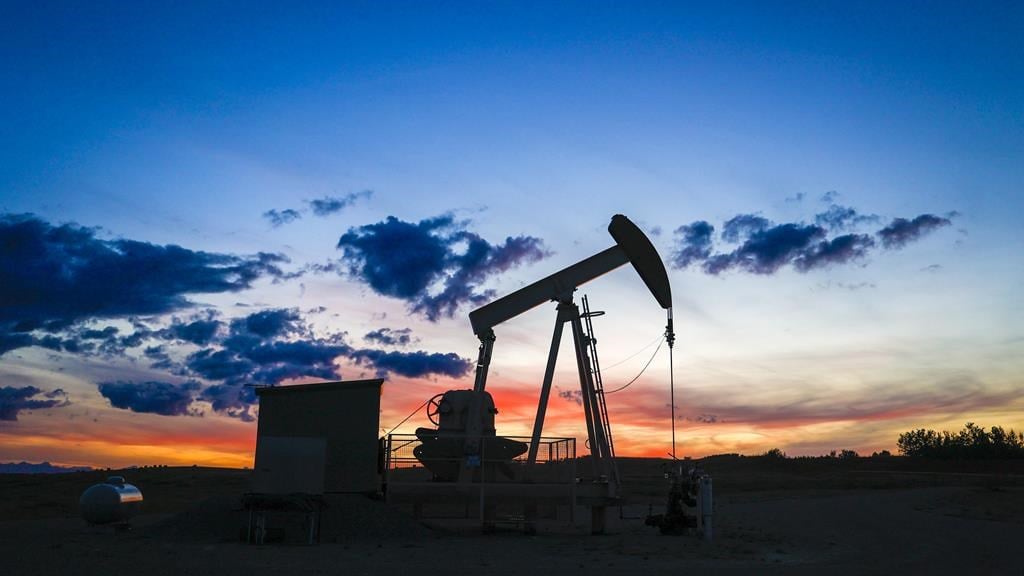In the serene dusk, a solitary oil pump stands as a silhouette against a vivid, multicolored sunset in a gently sloping field. The pump features a prominent hammer-like structure atop a platform, with metal wires cascading downward. To its left, a small building with a slightly arched roof is accented by a steel tank. The ground beneath appears light gray, possibly dirt or sand. Shadows of a wooded area and distant mountains frame the left side of the image, marking the horizon. Above this tranquil landscape, the sky transitions from deep blue at the top to a blend of white, pink, orange, and yellow near the horizon. Patches of dark clouds further enhance the dramatic twilight ambiance.